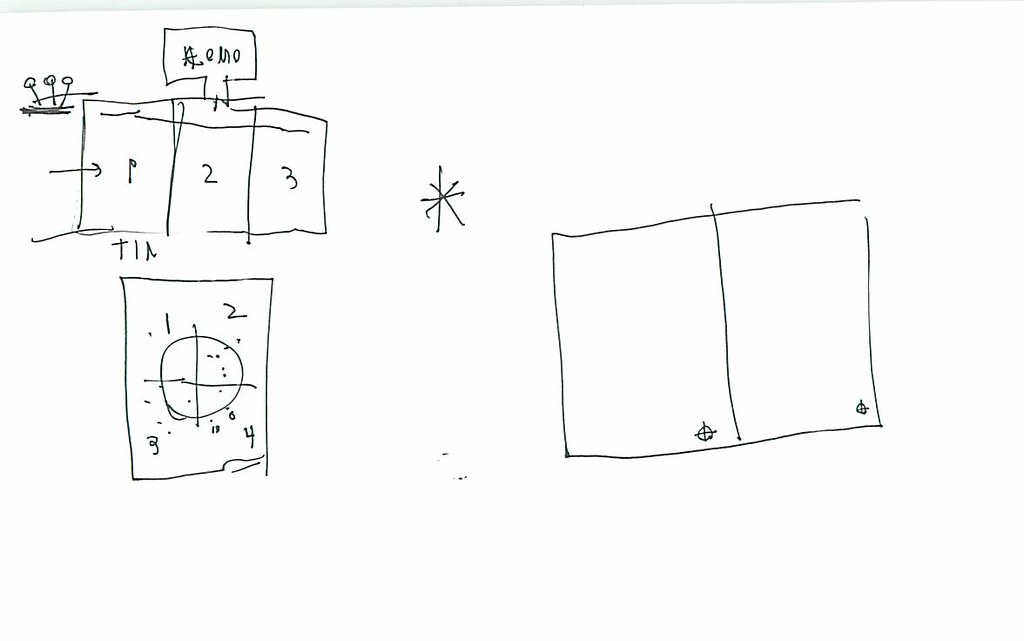This image showcases a detailed sketch on white paper, resembling a blueprint or conceptual plan. In the upper left corner, there are three connected rectangles labeled "1," "2," and "3" respectively. Above these rectangles, a rectangular sign that curves down to connect at the "2" reads "KOMO." To the left of this structure, three circles linked by vertical lines suggest the appearance of flowers or similar elements in the background.

An arrow points towards the rectangle labeled "1." At the bottom of the image, a larger rectangle contains a square with a central circle intersected by a plus sign, dividing it into four quadrants labeled "1" (top left), "2" (top right), "3" (bottom left), and "4" (bottom right). A star is prominently drawn at the center of the sketch. Additionally, on the right side of the image, two more rectangles feature a small circle with a plus sign in the corner.